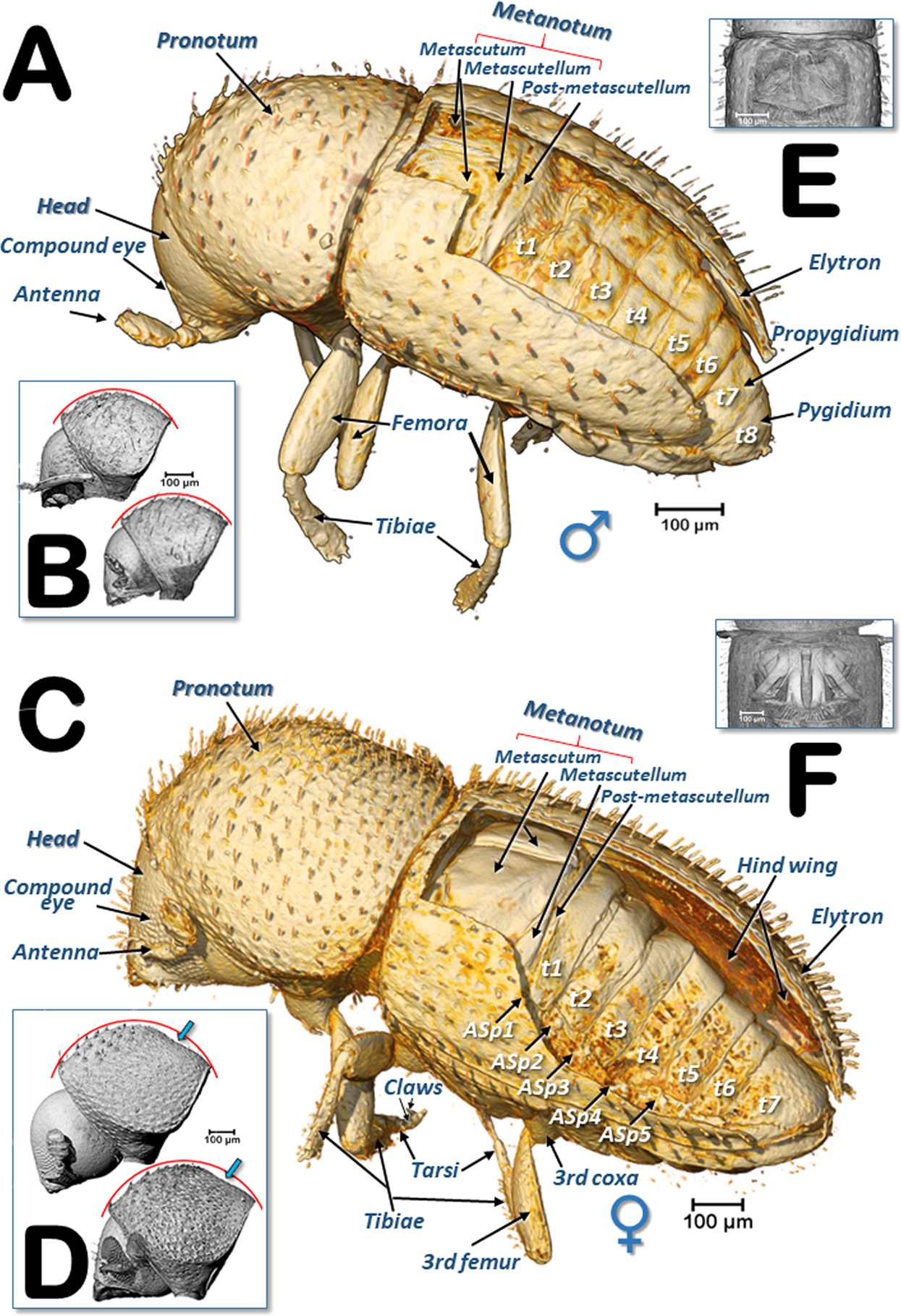This detailed diagram, likely from a scientific textbook, showcases two close-up, tan-colored insects, possibly belonging to the beetle or bed bug family. The drawing meticulously labels various parts of the insects with arrows pointing to significant anatomical features. The insects are divided into sections labeled A, B, C, D, E, and F, each highlighting different aspects of their anatomy.

The head section includes detailed labels for the head itself, compound eyes, and antennas. The body parts are labeled with terms like pronotum, metanotum, and elytron, while the back end of the abdomen features labels for the propygidium and pygidium. The legs are annotated to show the femora (femurs) and tibiae (lower leg segments), illustrating the insect’s complex structure. Additionally, the claws and hind wings are also detailed, with the hind wings particularly highlighted.

Inset labeling provides zoomed-in views of certain parts: inset A presents a detailed look at the outer parts of the insect, while inset B offers a close examination of more intricate features, potentially including the mouthparts.

The diagram includes both male and female specimens, clearly distinguished by their respective gender symbols. While both share similar anatomical structures, minor differences are noted, such as specifically labeled claws and hind wings on the female. A scale marker indicates the magnified nature of the drawing, specifying a measurement of 100 micrometers, hinting that these could be microscopic insects.